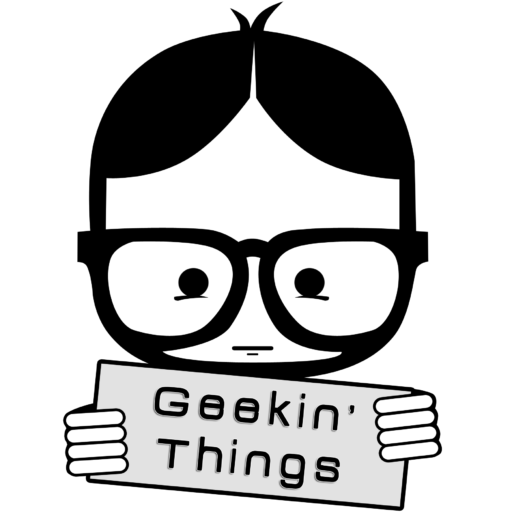The image is a detailed black and white drawing, likely intended as a logo, featuring a young man with a cartoonish appearance. His distinctive black hair is parted in the middle and styled with two prominent strands sticking up, resembling an alfalfa hairdo. He wears thick-rimmed, circular bifocals, which sit on his squarish round face, devoid of any real expression. His eyes are simple black dots with downward-curving lines underneath, and his mouth is a straight line with an additional short line below indicating the ridge of his bottom lip. He also has a very thin beard framing his chin. The character holds a rectangular gray sign, displaying the text "Geekin' Things" in black. Only his fingers are visible on either side of the sign, emphasizing the focus on the message he is presenting. The entire image is in grayscale, with the character drawn in black and white, adding to its minimalist yet nerdy aesthetic.